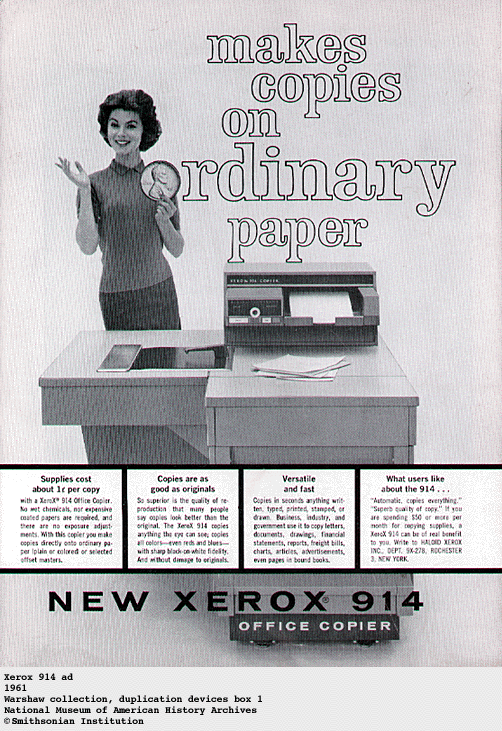This black and white 1961 advertisement for the Xerox 914, part of the Warshaw Collection at the National Museum of American History, Smithsonian Institution, features a smiling woman striking a pose reminiscent of a game show model. She holds up an oversized penny with her left hand, aligning with the text at the top that reads "Makes copies on ordinary paper," where the 'O' in "ordinary" is shaped like a penny. Standing behind a Xerox 914 office copier, the machine itself is prominent, showcasing a stack of paper. Bulleted points below highlight the copier's benefits: supply costs about 1 cent per copy, copies as good as originals, versatile, and fast. The ad, distinctly old-fashioned, emphasizes in bold letters at the bottom, "New Xerox 914 office copier," capturing the breakthrough of making copies on ordinary paper.